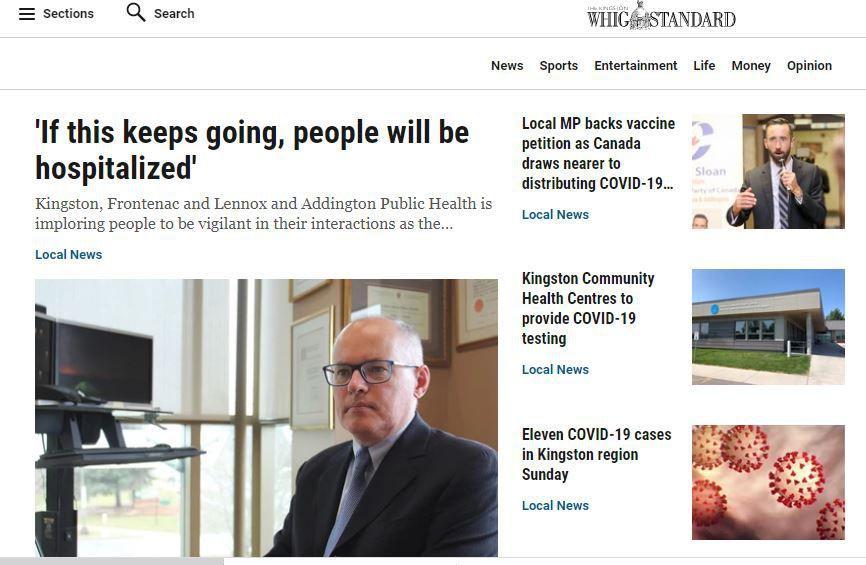The image is a screenshot of a news website titled "WIG Standard." The website's navigation bar at the top features various categories including News, Sports, Entertainment, Life, Money, and Opinion. Below the navigation bar, several article thumbnails are displayed.

On the left side of the page, the most prominent article is featured with the largest image and headline. The headline reads: "If this keeps going, people will be hospitalized." The article is about Kingston, Frontenac, and Lennox and Addington Public Health urging people to be cautious in their interactions. The accompanying image is of a white man wearing glasses and a suit, likely a health official or professional based on the context of the headline.

Adjacent to this main article are smaller articles with brief headlines and thumbnails. One headline states, "Local MP backs vaccine petition as Canada draws near to distributing COVID-19 vaccines." Another article is titled, "Kingston Community Health Centres to provide COVID-19 testing." The final headline reads, "11 COVID-19 cases in Kingston region Sunday." All these articles fall under the local news category.